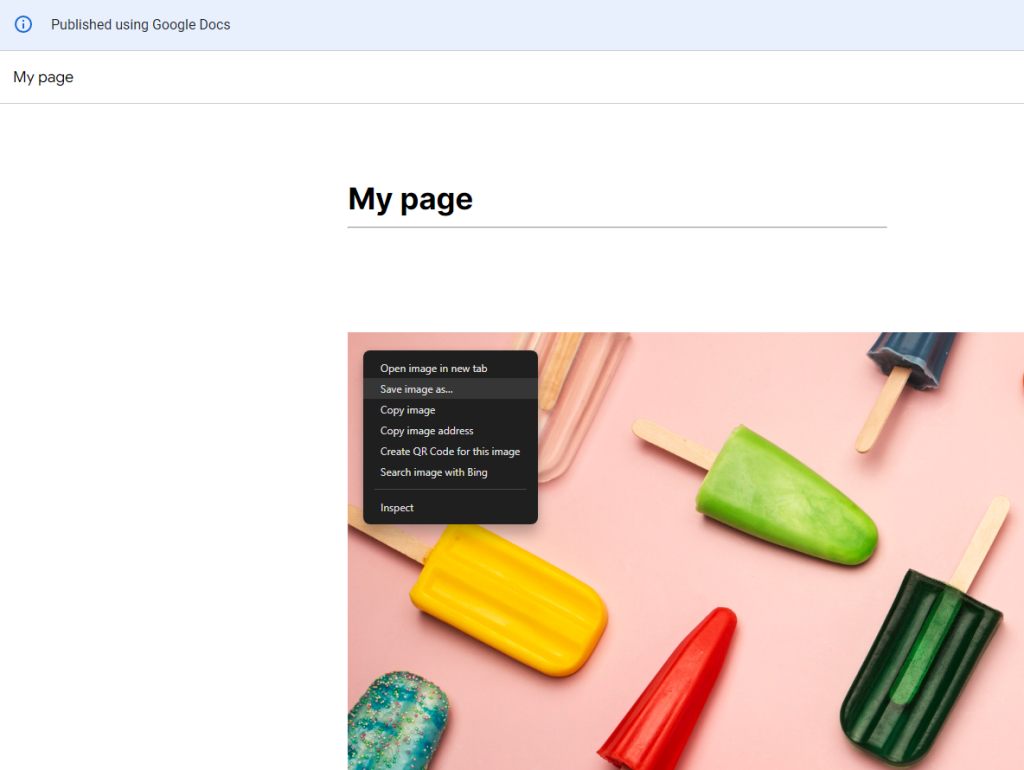This color screen capture displays a webpage with a predominantly white background. At the top of the screen, a blue bar stretches horizontally, bearing the text "Published using Google Documents" in white. Beneath this, the text "My Page" appears in black, followed by a black horizontal line. Centrally positioned, "My Page" is written again in a bolder, darker black font, underlined with another black line.

The background of the page showcases an assortment of colorful popsicles lying flat on sticks, set against a pink backdrop. The popsicles are organized in an array of vibrant colors, including yellow, red, light green, dark green, blue, light blue, and clear. Notably, the blue popsicle in the bottom left corner and the darker blue one in the top right corner are mostly out of frame.

A black drop-down menu is prominently displayed on the right side, listing options such as "Open image in new tab," "Set image as," "Copy image," "Copy image address," "Create QR code for this image," "Search image with Bing," and "Inspect." The text in the drop-down menu is white, contrasting with the black background, and the option "Save image as" is highlighted.